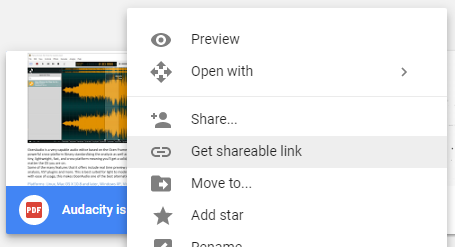The image displays a partial screenshot of a Google Drive interface, characterized by Google’s distinct icons and fonts. In the background, a PDF thumbnail with its title and format is visible. In the foreground, a pop-out menu is present, listing several options: "Preview," "Open with" (indicated by a right-facing arrow), "Share," "Get shareable link," "Move to," "Add star," and "Rename," with each option accompanied by a corresponding icon. The "Get shareable link" option is highlighted in dark gray, suggesting it is currently selected. Notably, the bottom part of the image appears to be cut off, implying that only about 50% of the screenshot is visible, potentially concealing additional details.